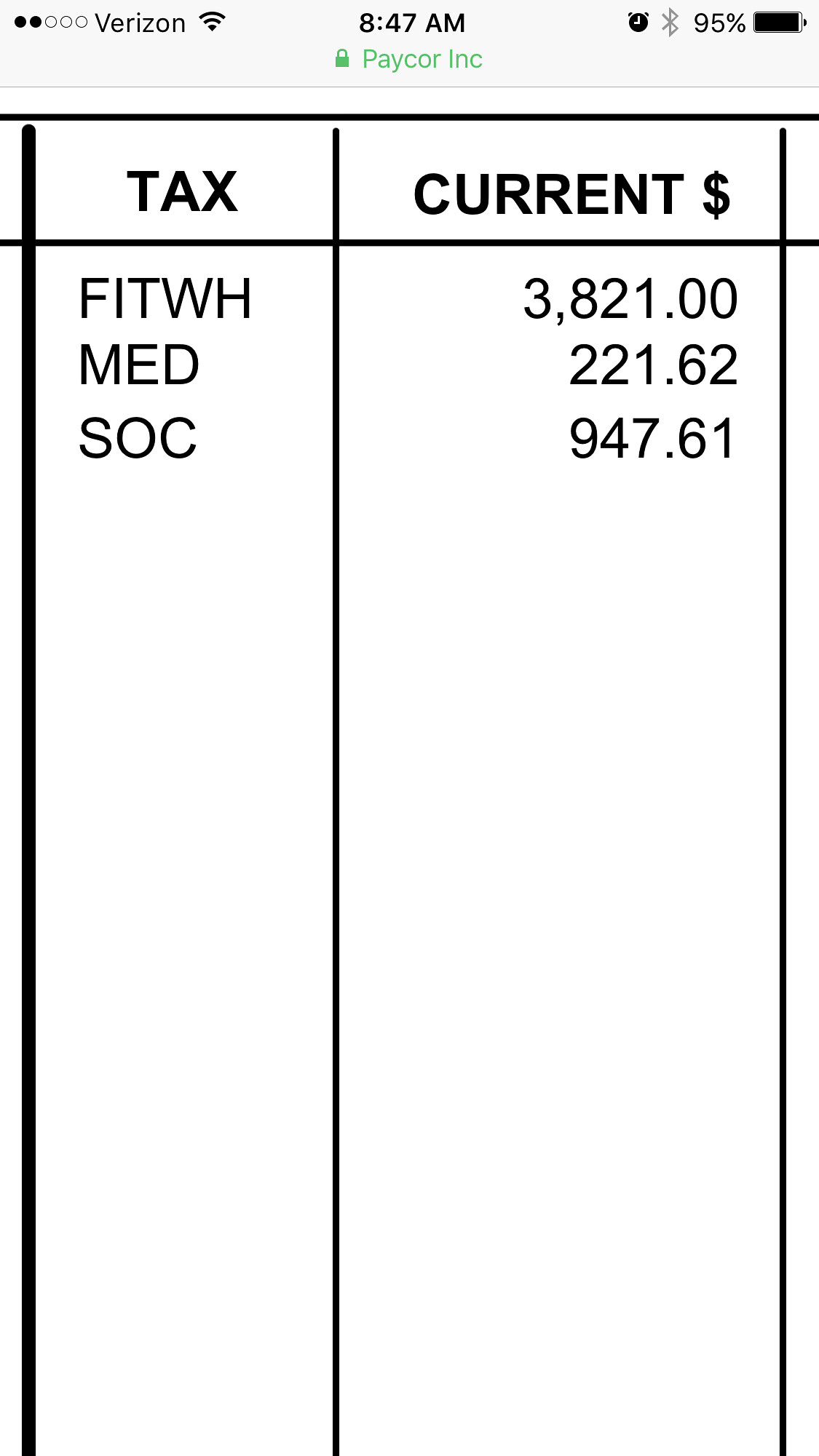This is a mobile screenshot from a Verizon phone, displaying a transaction summary. At the top, the status bar includes the Verizon logo, the time "8:47 AM," the Wi-Fi icon, and a battery indicator showing 95% charge. Beneath this, in green letters, it says "Paycor Incorporated" with a green lock icon next to it, indicating a secure connection. The main section of the screenshot is organized into two columns. The left column is titled "Tax" and contains three items: "FITWH" indicating Federal Withholding Tax, "MED" for Medicare, and "SOC" for Social Security. The corresponding amounts are listed in the right column under "Current $": "$3,821.00" for FITWH, "$221.62" for Medicare, and "$947.61" for Social Security. This detailed mobile screenshot appears to summarize payroll tax deductions.